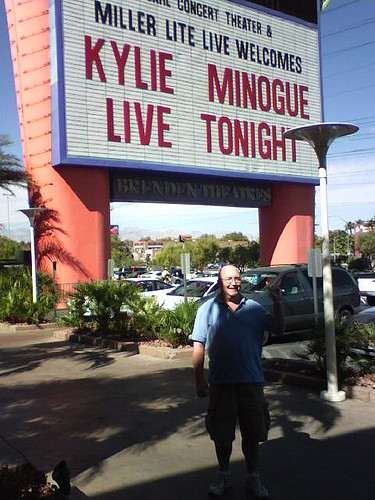In this vibrant photograph, an older man wearing eyeglasses stands outside on a sunlit sidewalk, smiling warmly. He is dressed casually in a blue polo shirt, cargo shorts, and white shoes. The setting is lively and urban, marked by tropical greenery in the medians where sidewalks converge, and tall, green palm trees that sway gently in the breeze. Overhead, the sky is a brilliant blue sprinkled with a few white clouds, hinting at the warmth of the day.

Dominating the scene behind the man is a massive sign that reads, "Miller Light Live Welcomes Kylie Minogue Live Tonight." Below this prominent sign, another sign with the name "Brendan" adds a personal touch to the bustling backdrop. The man is partially shaded by objects in the area, casting intriguing patterns on his figure. The surrounding area is composed of asphalt and is adorned with white light poles and power lines that trace the sky in the distance.

Behind him lies a sprawling parking lot filled with cars, emphasizing the busy nature of this lively concert event. To complete this lively urban scene, the background also features a distant view of numerous trees, adding a touch of nature to the dynamic cityscape.